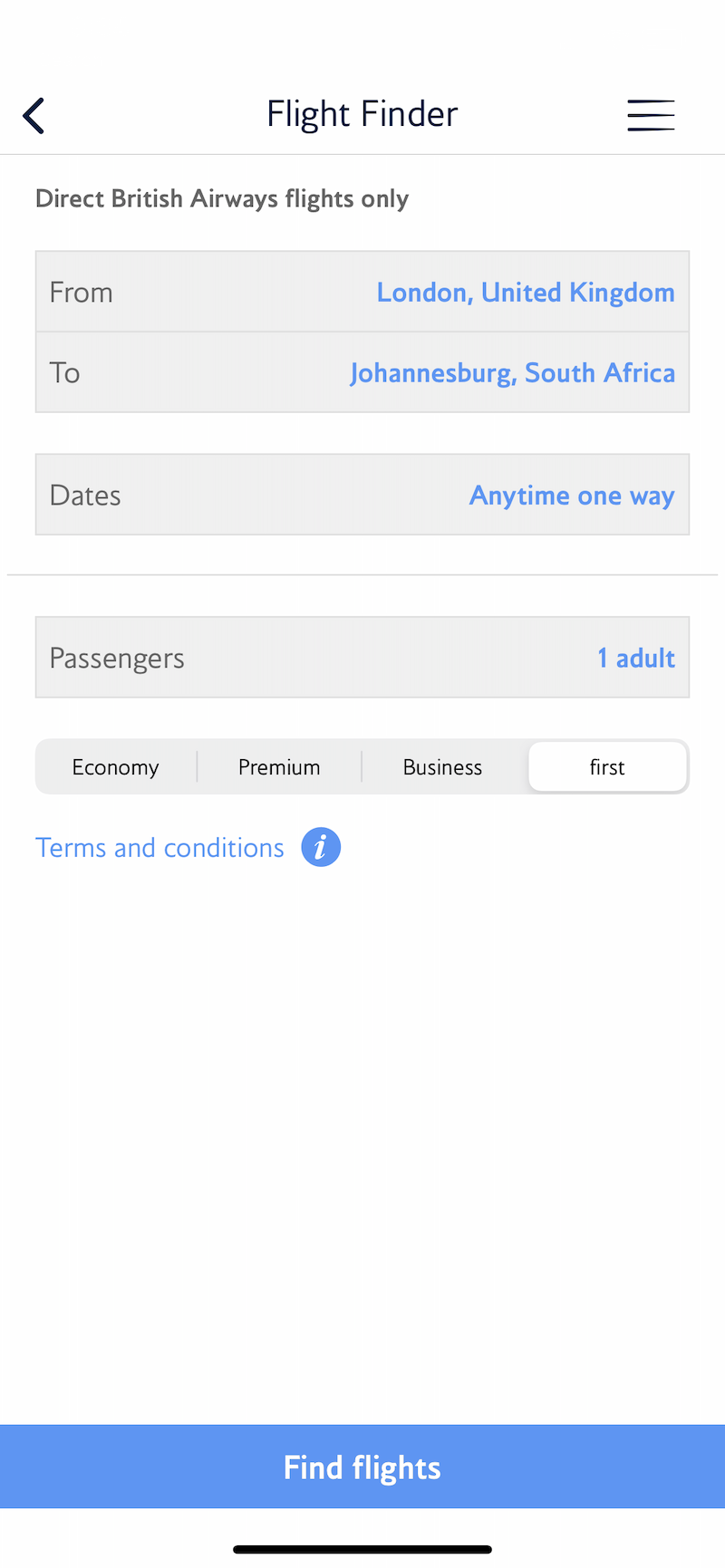Here is a cleaned-up and detailed caption for the described image:

"Displayed is an online flight search interface for booking flights from the United Kingdom to Johannesburg, South Africa. At the top center, there is a flight finder tool flanked by a back arrow on the left and a settings icon on the right. Below, a checkbox labeled 'Direct British Airways flights only' is visible. 

The main section contains input boxes for flight details: the 'From' box is on the left, showing 'London, United Kingdom' in blue on the right side of the box, and directly below it is the 'To' box indicating 'Johannesburg, South Africa' also in blue. Users can specify travel dates in another section labeled 'Dates: Anytime' and choose between one-way or round-trip with toggle options. 

There is a 'Passengers' box displaying '1 Adult' in blue, and next to it, the current selected class is 'First Class,' with options to switch to Business, Premium Economy, or other cabins. 

Terms and accommodations information is provided beneath these options, highlighted in blue, with an information icon ('i') for further details. At the bottom of the interface, a prominent blue 'Find Flight' button invites users to initiate the search after inputting all necessary parameters such as origin, destination, travel dates, and number of passengers."